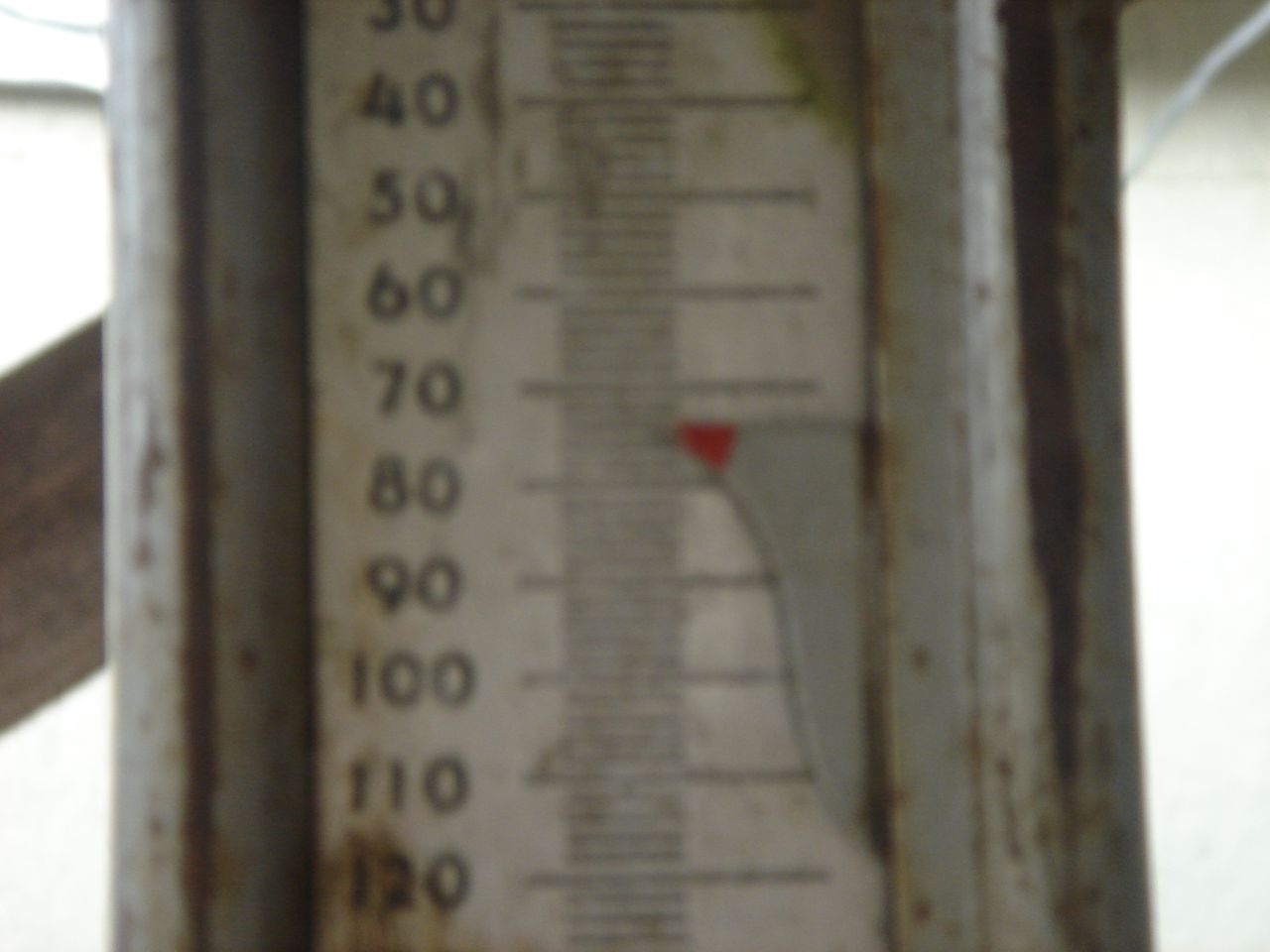The image features an aged, silver outdoor thermometer mounted against a backdrop of white baby siding. The siding appears weathered, complementing the rustic aesthetic of the scene. To the left, dark wood grain adds a contrasting texture to the composition. The thermometer itself is heavily tarnished and rusted, showcasing a mix of deep black corrosion and yellow-gold rust in various areas, evidencing prolonged exposure to the elements. Despite the wear, the thermometer's numerical range from 30 to 120 degrees is still visible, albeit through a layer of dirt. The red pointer is positioned around 75 to 85 degrees. The metal casing of the thermometer displays scratches, contributing further to its weather-beaten appearance.